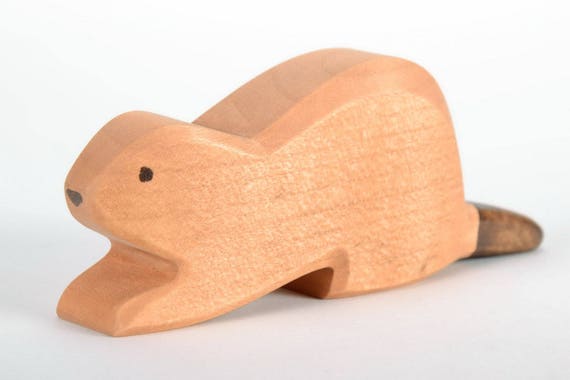The image captures a finely sanded, carved wooden sculpture depicting a small animal, most likely a beaver, given its characteristic features. It has a natural wood color, except for the tail, which is stained a darker shade, and subtle stains to highlight its nose and eyes. The animal is positioned on its tummy with its front and back legs extended out, treated as single, undivided sections for each pair of limbs. The simple yet endearing sculpture is finished with a sleek, shiny coating, perhaps polyurethane, giving it a smooth, water-resistant surface. The background of the rectangular image transitions from pure white at the top to a gradient gray at the bottom, directing all focus to the beaver figure.